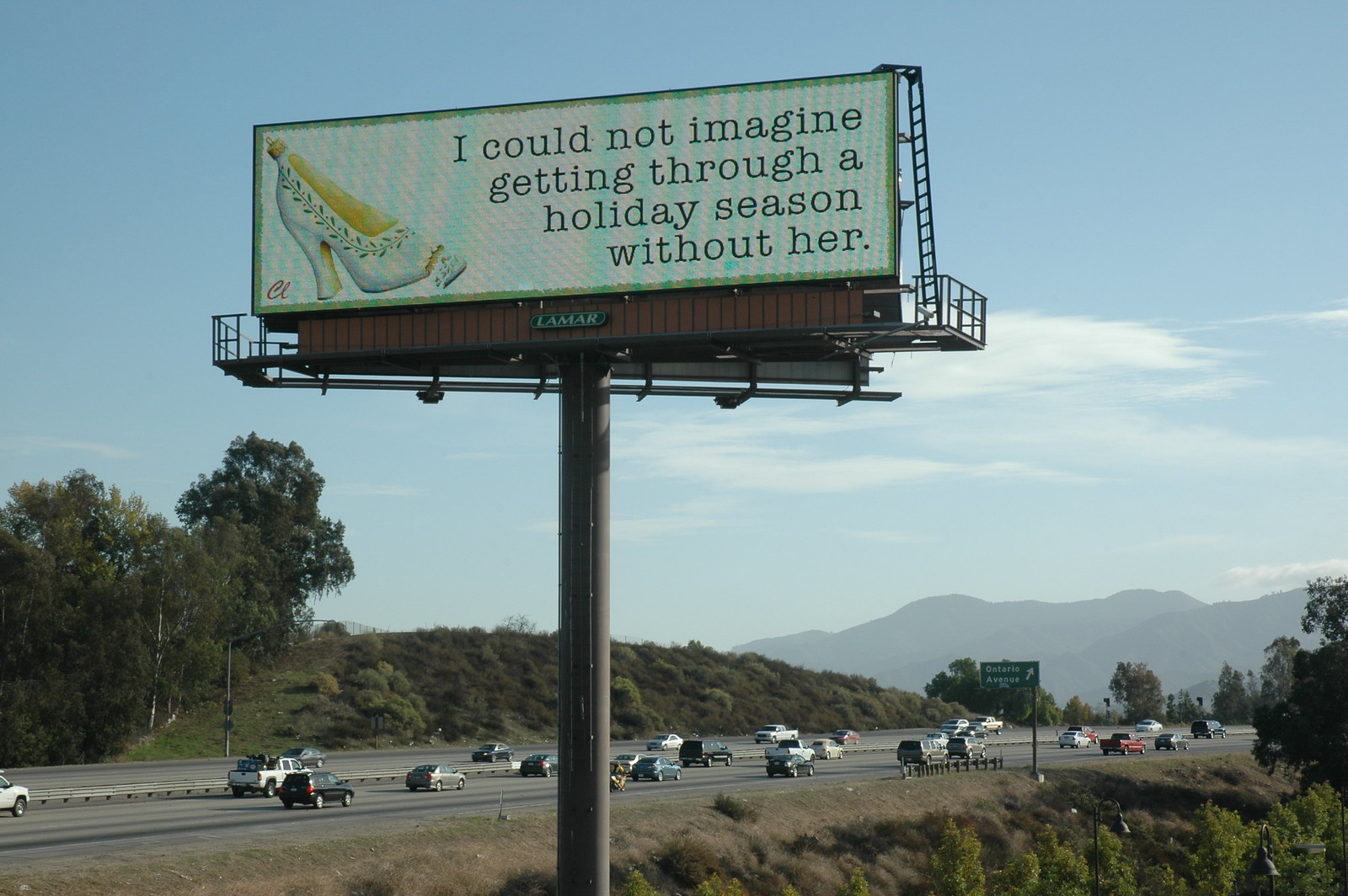This photograph captures a large billboard prominently situated in the center of the frame. The billboard is supported by a dark brown metal structure and features a clean, white rectangular canvas bordered by a vibrant lime green outline. The text on the billboard is in stark black and reads, "I could not imagine getting through a holiday season without her." To the left side of the advertisement, there is an intriguing bottle designed to resemble a high-heeled shoe. This high-heeled shoe bottle is entirely white, adorned with green leaves around the opening where one would typically insert their foot. In the background, a major gray highway stretches across the landscape, flanked by verdant hills covered in lush green bushes and interspersed with mature trees, all fully outfitted in green foliage. The overall scene presents a harmonious blend of commercial messaging and natural beauty.